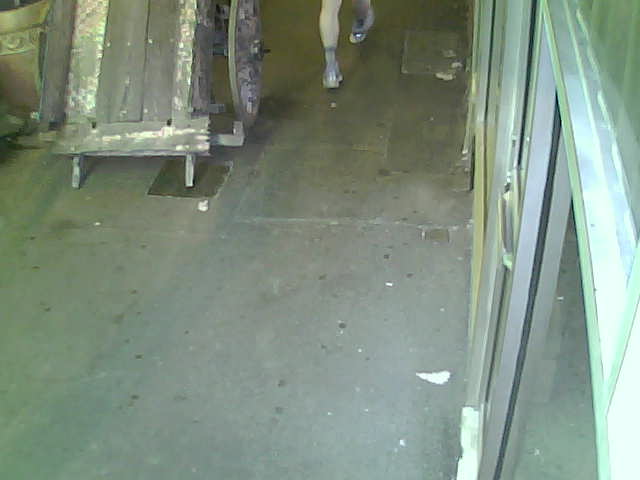This photograph captures a work area characterized by a well-worn concrete floor, stained and spotted from years of use. In the upper left corner stands a vintage wooden cart, distinguished by its old-fashioned wooden wheels and metal brackets. The cart's surface is heavily worn, suggesting it has been used extensively for heavy pulling and moving tasks, possibly within an open market or auction setting typical of a traditional fish market in Far East Asia, such as Japan. Additional carts visible in the scene also hint at their use for transporting goods within a warehouse or market area. On the right side of the image, a metal window frame is visible, through which natural light filters. In the uppermost part of the image, just above the frame, the legs and feet of an individual wearing shorts can be seen, adding a human element to this snapshot of a bustling, historically rich work environment.